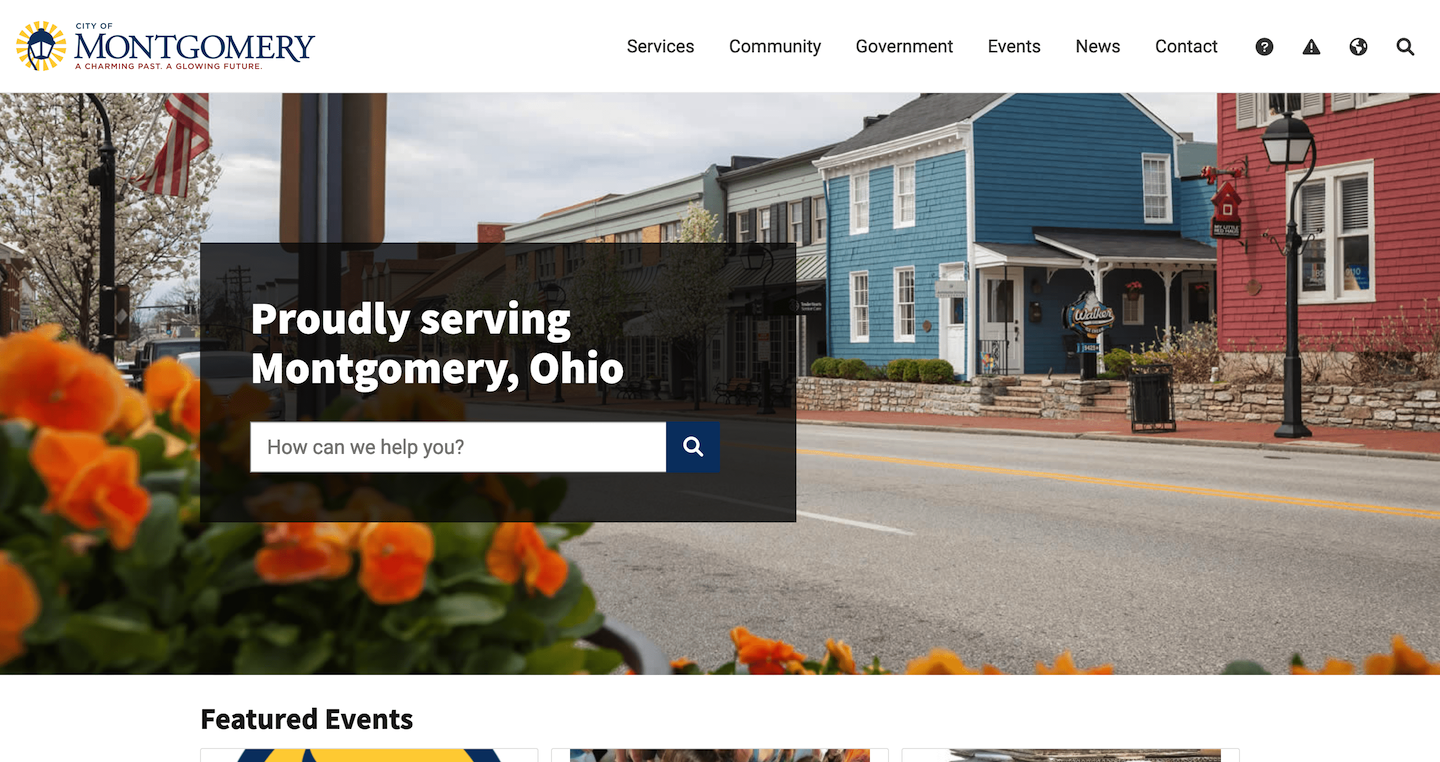This image appears to be a screenshot of a website focused on the City of Montgomery, Ohio. The primary section of the image showcases a picturesque neighborhood landscape. On the right side and stretching across the top of the screen, several homes are visible. To the left, an assortment of colorful flowers and dense shrubs lines the street. A road separates the houses from the foliage, bordered by trees and additional greenery.

Superimposed over this serene scene is a semi-transparent text box that reads, "Proudly serving Montgomery, Ohio." Below, a white search box invites users with the prompt, "How can we help you?"

At the very top of the image, the header contains the city's branding elements. On the left, the text "City of Montgomery" is accompanied by a yellow and blue logo resembling a street lamp, accompanied by the motto, "A Charming Past, A Glowing Future." To the right, a navigation menu offers links labeled Services, Community, Government, Events, News, and Contact, along with several icons including a search icon and possibly a map icon, among others.

Finally, at the bottom of the image, beneath the landscape photograph, there is a section titled "Featured Events," which displays three partially visible event images.